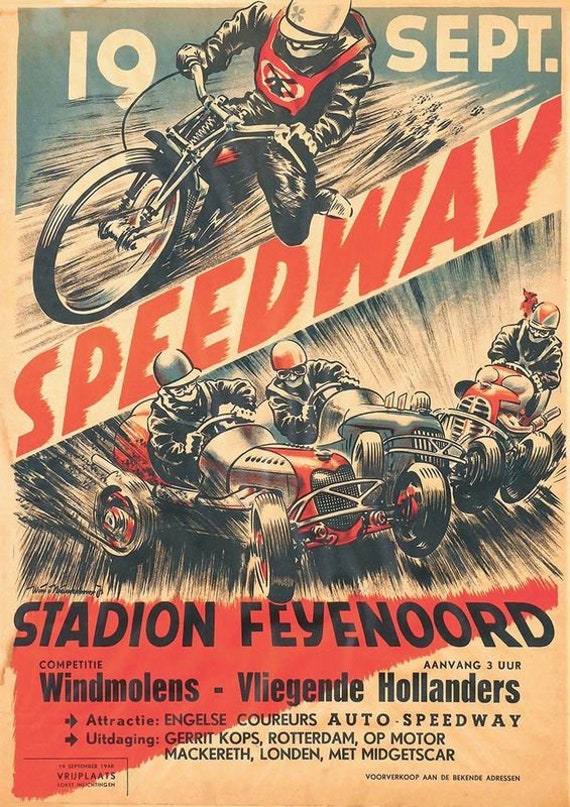Advertisement poster for a vintage race event held at Stadion Feyenoord, located in the Netherlands. The event date, "19 September," is displayed at the top against a light blue background in bold white text. Furthermore, the prominent title "Speedway" is emblazoned across the center in striking red. The upper section of the poster features an animated illustration of a man riding a motorcycle, adorned in a red vest and white helmet. Below, three classic open-hooded cars driven by helmeted men are depicted, capturing the essence of a bygone era with their nostalgic charm. The bottom section is highlighted in red with black text that reads, "Stadion Feyenoord," detailed further with Dutch terms, "Vindmolens, Willeganda, Hollanders," enriching the poster with local flavor. The overall color scheme suggests an aged, yellowish-brown paper, enhancing the vintage aesthetic of this compelling race advertisement.